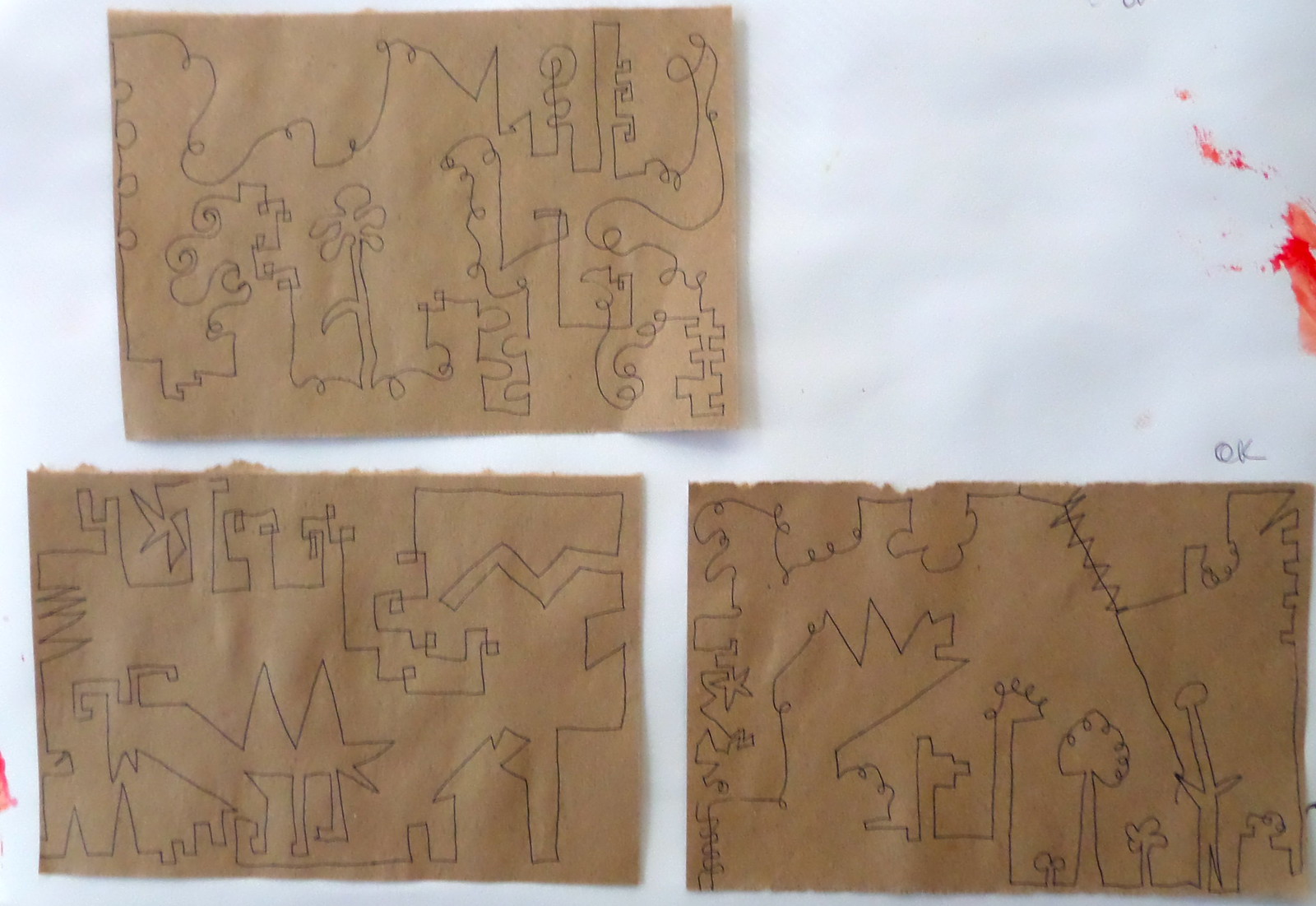The image showcases an abstract work of art on a white background, reminiscent of finger paint paper. Scattered in the upper right and lower left corners are subtle splotches of red and orange paint. Dominating the scene are three torn rectangles of brown paper, akin to repurposed shopping bags, affixed to the white surface. The rectangular pieces are uniquely positioned — two neatly placed at the bottom, and one situated in the upper left corner, slightly askew, leaving some white space visible. Each brown rectangle is adorned with intricate black pen line drawings, featuring continuous, unbroken lines that meander in loops and various shapes before returning to their starting points. The first drawing is characterized by fluid squiggles, the second by sharp angles, and the third by a combination of both styles. The image maintains a simple yet evocative color palette of white, black, brown, red, and orange, suggesting a setting possibly within an indoor elementary classroom.